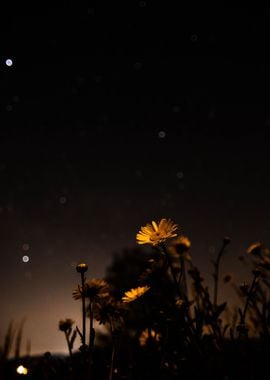This vertical, low-resolution nighttime photograph captures a close-up view of yellow flowers, possibly daisies or dandelions, bathed in an eerie yellowish glow. Two open flowers take prominence in the foreground, surrounded by small buds and additional flowers scattered in the background, creating a clustered, delicate scene as they grow out of the ground. The image conveys a dreamy, almost ghostly atmosphere, accentuated by a gradient that transitions from the warmly lit bottom to a black sky overhead. Distant stars or bokeh-like circles pepper the sky, adding to the ethereal quality. A faint moonlight glow appears near the horizon, casting subtle light on the flowers and creating silhouettes from those further back, offering a striking contrast between the illuminated petals and the dark field.